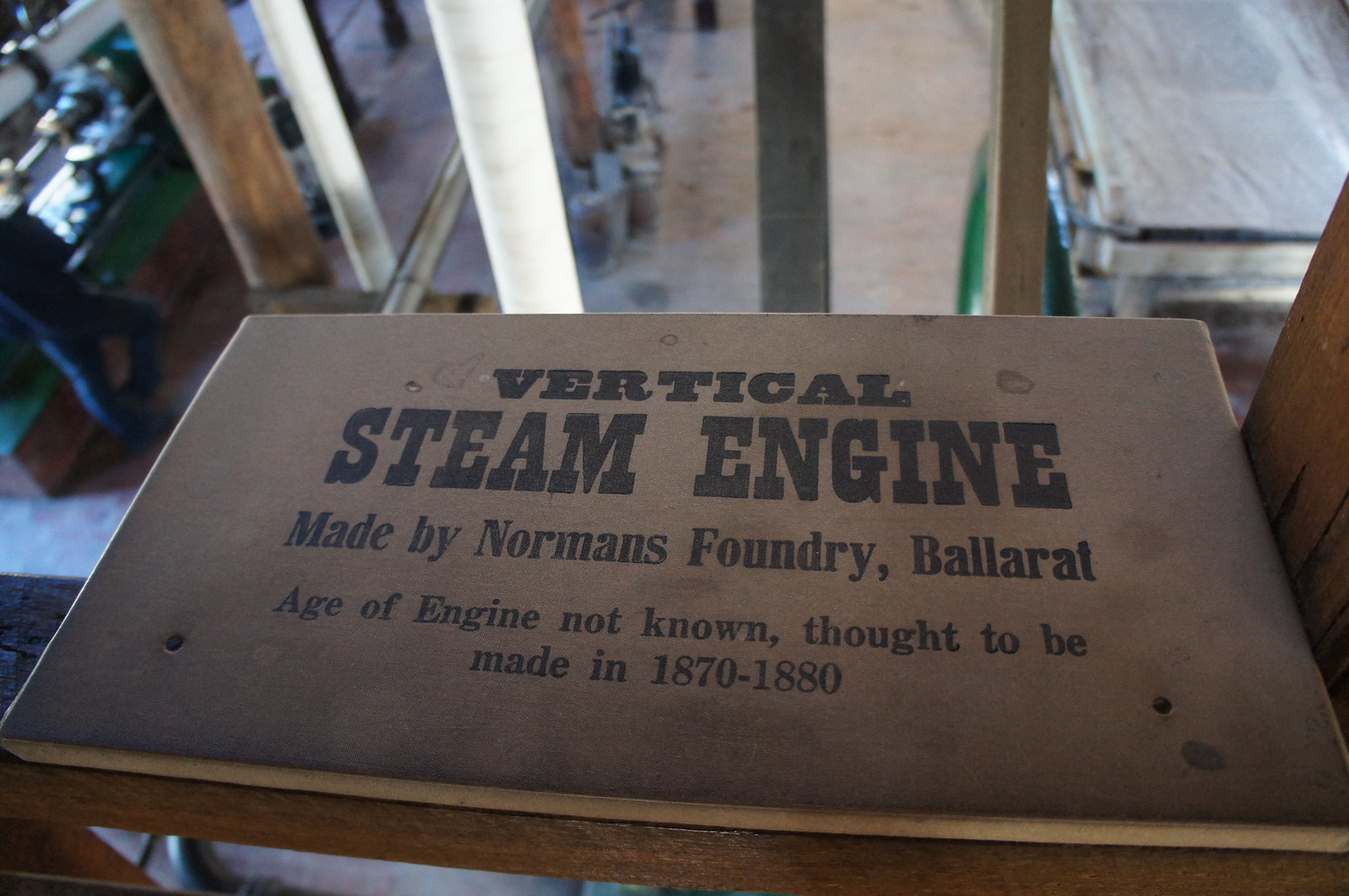The photograph captures a wooden plaque fastened to a railing on an elevated second-floor vantage point, overlooking a spacious facility, possibly a factory or warehouse. The plaque, styled with vintage 1800s text, reads: "Vertical Steam Engine. Made by Norman's Foundry, Ballarat. Age of the engine not known. Thought to be made in 1870 through 1880." Although the steam engine itself is not visible from this angle, the background reveals machinery and industrial equipment, hinting at the site's dedication to mechanical history or restoration. A figure is partially visible on the left, and the distant floor emphasizes the photograph's high vantage point. The scene is well-lit, highlighting the plaque and hinting at a space filled with historic industrial artifacts, including what appears to be an old car or truck covered with a tarp, suggesting ongoing restoration work.